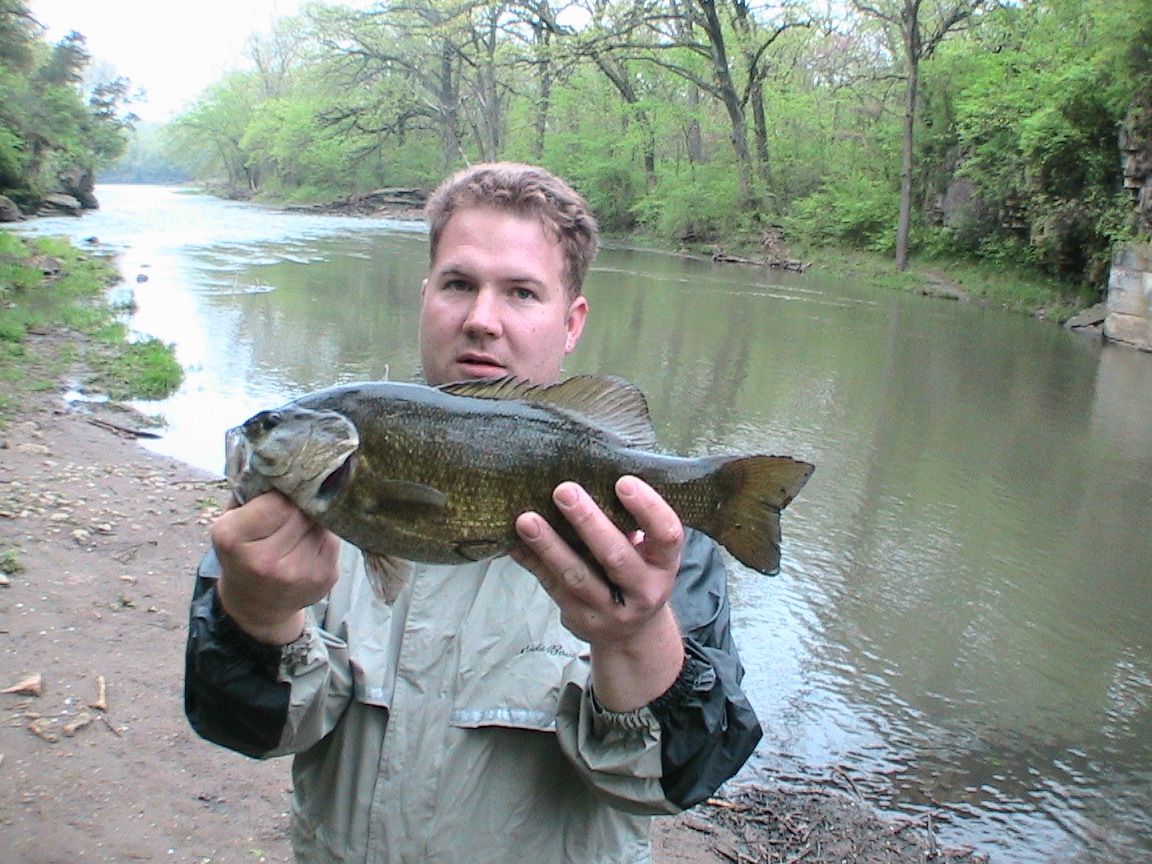In this outdoor photograph, a young white man with light brown hair, appearing to be in his thirties, stands at the muddy, rocky edge of a coastline. He is wearing a light gray and dark gray rain jacket, holding a greenish-gray fish in each hand, proudly presenting them towards the camera. The background reveals a large body of water, likely a river due to its murky and muddy appearance, flanked by lush green trees and shrubs. The atmosphere is characterized by a cloudy sky, indicating it's an overcast day.